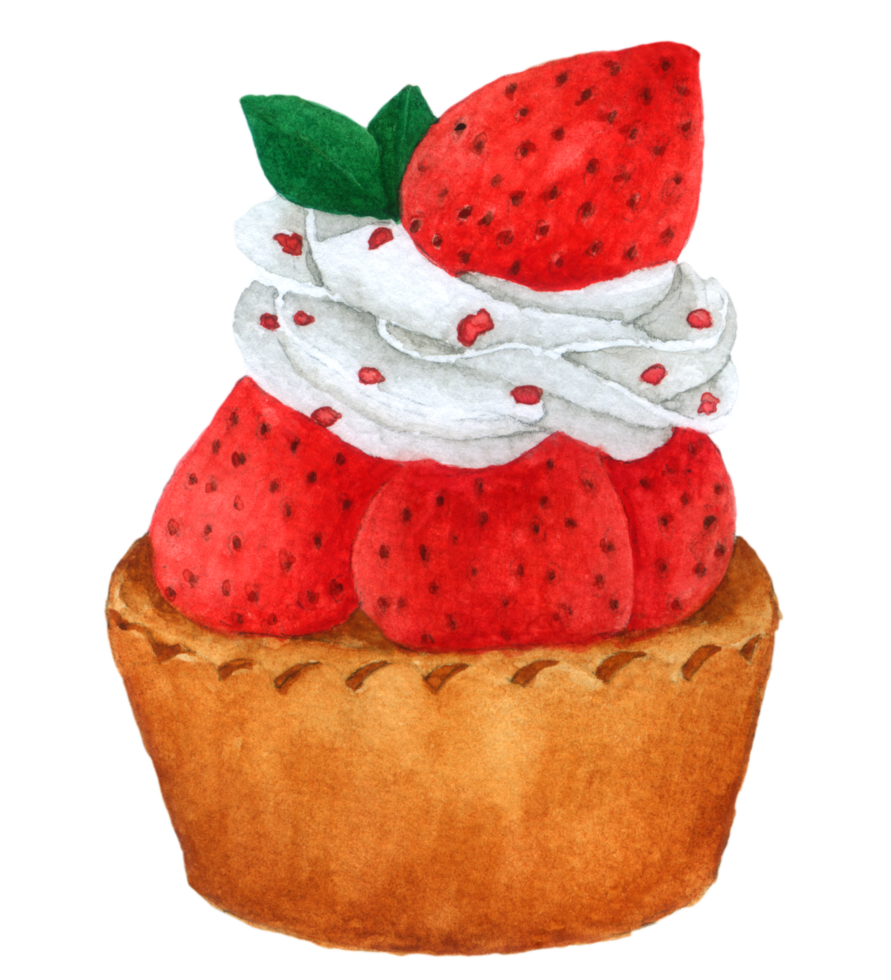In the image, there is a large, detailed drawing of a delectable dessert, likely a strawberry shortcake or cupcake. The base of the dessert is a light brown, tan color, giving the impression of something like a cupcake wrapped in a matching light brown wrapper or parchment paper, complete with scalloped edges. The base takes up about a third of the image and appears to be light and fluffy, possibly angel food cake or yellow cake.

Above the base, there are three whole, uncut strawberries, vibrant red in color, perfectly arranged. Crowning these strawberries is a generous dollop of white whipped cream, speckled with tiny red dots, potentially finely chopped strawberries or decorative sprinkles. 

At the very top of the dessert sits a large, prominent strawberry, the tip of which points slightly to the right. This top strawberry is accompanied by two small, green leaves, likely from the strawberry plant or perhaps mint, adding a fresh and colorful garnish. The entire dessert is set against a clean, white background, making the vivid colors and intricate details of the dessert stand out beautifully.